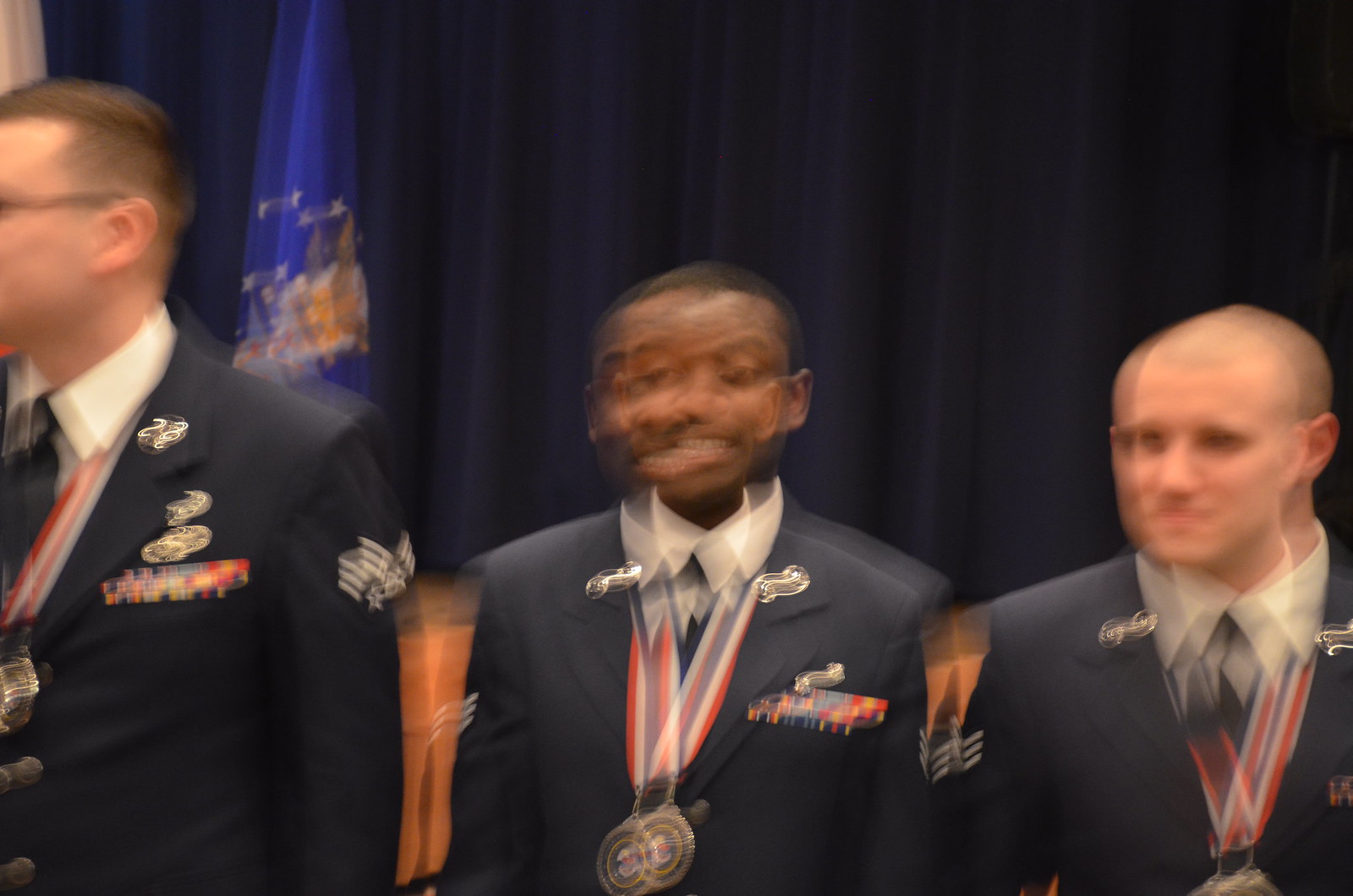In this extraordinarily blurred image, three men are standing proudly, each adorned with medals featuring red, white, and blue ribbons. They are clad in dark military uniforms, exuding a sense of honor and achievement. The man on the left, as observed, is notably taller than the other two. The trio stands against a backdrop that appears to be an auditorium stage, embellished with what seems to be a dark blue curtain. To the side, a U.S. departmental flag is visible, characterized by an eagle with outstretched wings set against a royal blue background, likely linked to the Department of Defense or a similar governmental body. Despite the image's lack of clarity, the palpable joy and pride on the recipients' faces shine through, capturing a moment of significant recognition and celebration.